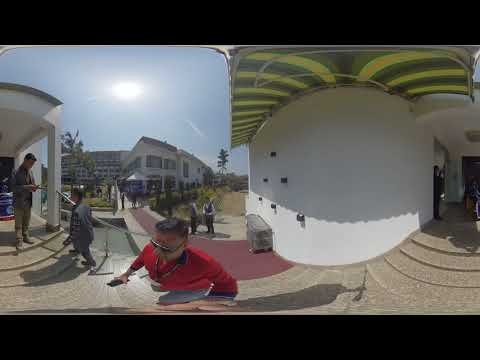In this vibrant outdoor scene, we see a man in a red shirt and blue pants walking away from a white building under a clear, almost cloudless, light blue sky. Captured from a top-down perspective, he wears sunglasses and is holding something in his right hand. The setting appears to be a sunny day on a college campus or an office complex, with the bright sunlight casting distinct shadows. The building has a unique wraparound design with few brown cobblestone steps and a green-and-yellow striped ceiling cover, possibly resembling a courtyard or an archway leading to different areas. 

To the left of the man, two others are near shallow steps; one individual is ascending them into the white building, while another stands at the top in conversation. A few stories-high, wide, round white building stands prominently in the background, bordered by grass, trees, and sidewalks where a couple of additional people are visible. The scene also features a hallway with steps leading up to what looks to be an office area, and various architectural elements suggest this could be a hotel, apartment complex, or even a country club. The photo, potentially taken with a fisheye lens, melds multiple perspectives into one cohesive image.